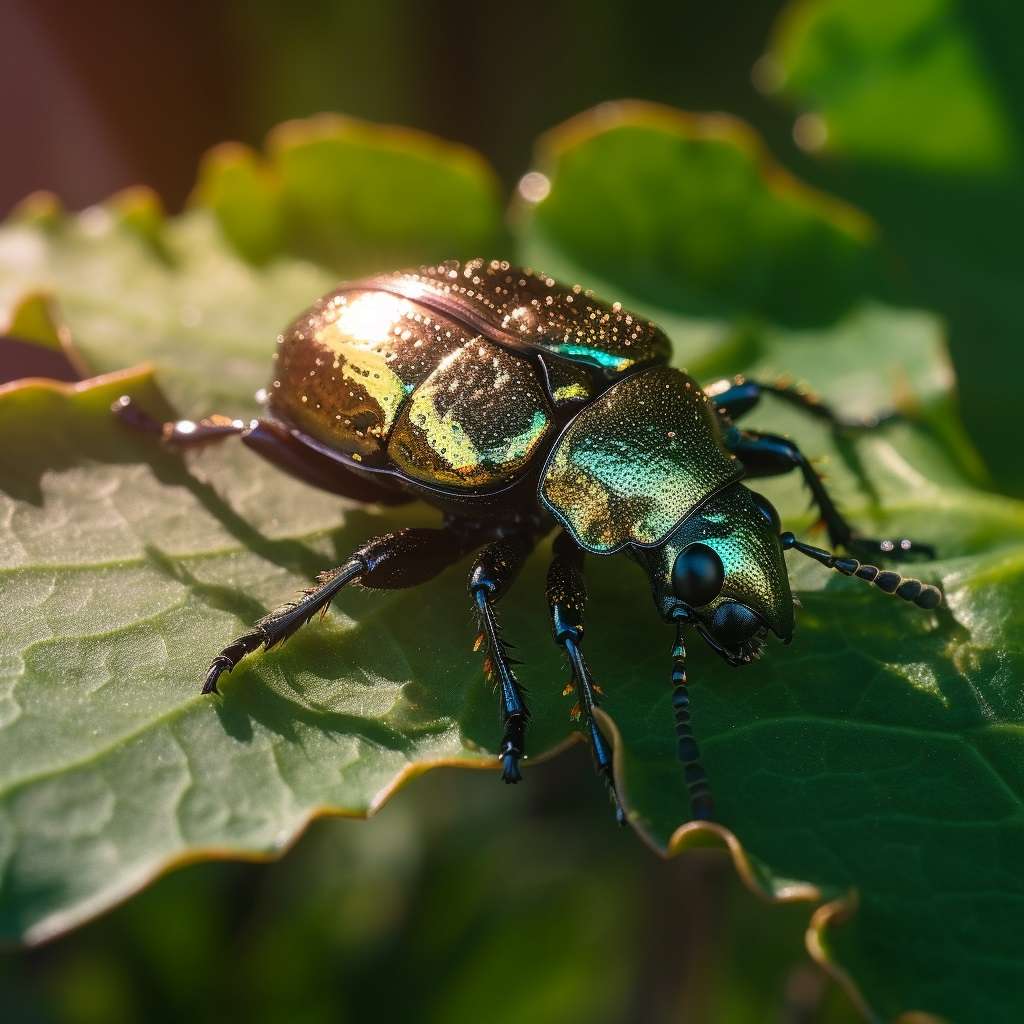The full-color photograph captures a vibrant, close-up shot of a multicolored beetle perched on a leaf, taken outdoors on a sunny day. This professionally done artistic nature shot is horizontally rectangular with no visible border. The background is a blurred green, hinting at foliage but remaining indistinct. To the left, sunlight streams down, illuminating both the leaf and the beetle, which serves as the primary focus of the image. The beetle, characterized by its hard, shiny shell adorned with a mesmerizing mix of yellow, green, black, purple, and red hues, also features tiny droplets of moisture scattered across its exoskeleton. The beetle displays long antennae, black eyes, and four prominent eyes on its head. The insect possesses six somewhat hairy black legs, emphasizing its distinctive beetle shape.